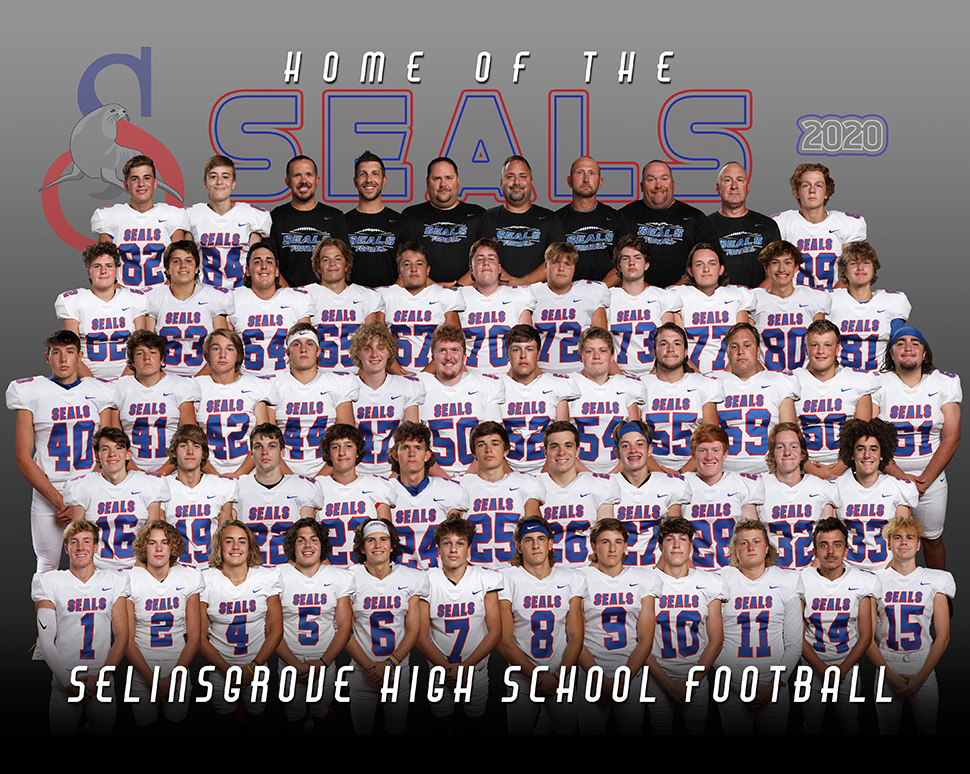This image is a meticulously composed team poster for the Sullins Grove High School football team, prominently featuring the phrase "Home of the SEALS 2020" in large, eye-catching text at the top. The word "SEALS" is crafted in a vibrant blue bubble font with a gray fill and red outline, also accompanied by a distinctive logo in the top left corner of a seal enclosed by a large, color-divided "S" in blue and red. The background transitions from light gray at the top to black at the bottom, providing a sleek backdrop that highlights the team. The team members, over 50 in total, are arranged in five neat rows. The bottom four rows are comprised entirely of high school boys in white SEALS jerseys with blue numbers and red outlines. The top row includes three players at either end and seven coaches in the center, distinguishable by their black T-shirts emblazoned with the SEALS logo in blue. At the bottom of the image, in white capital letters, it reads "SELINSGROVE HIGH SCHOOL FOOTBALL," completing this comprehensive team portrait.